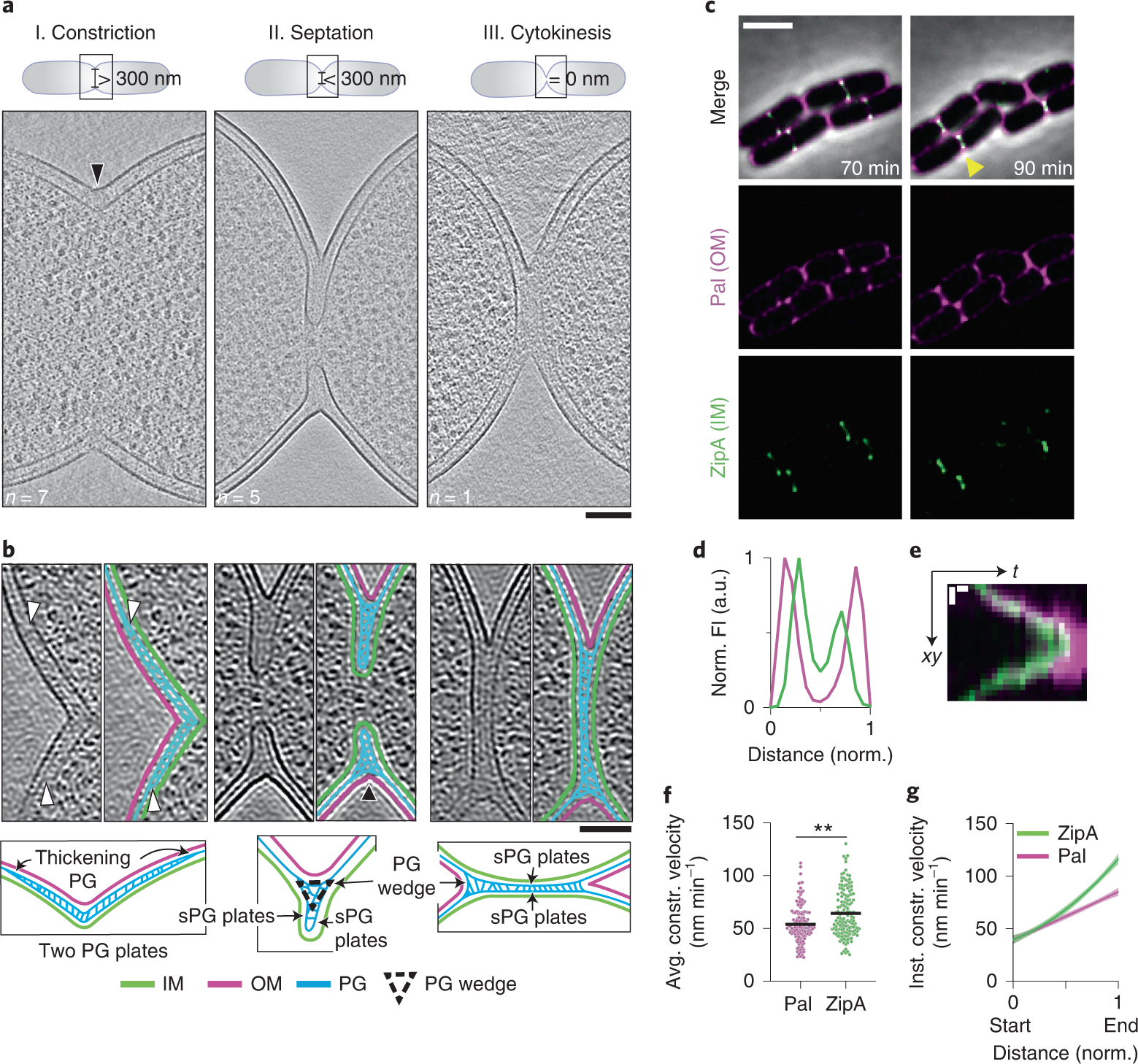The image displays a detailed scientific analysis on a white background, beginning with labeled sections "A" through "D." The top part of the image features a series of six microscopic photographs of cells undergoing various stages of division: constriction, septation, and cytokinesis. Below these pictures, there are additional images showing tissue with wedges and thickening PG with SPG plates. On the right side of the image, data focuses on constriction velocities, norm distances, and start-to-end distance measurements, characterized with graphs that display changes over time, noted at intervals like 70 and 90 minutes. The graphs also include labels such as 1 (normal) and show distances up to 150 units, highlighting a critical data point at 48. The images and figures collectively illustrate the progressive changes in cellular structures under different conditions and timeframes.